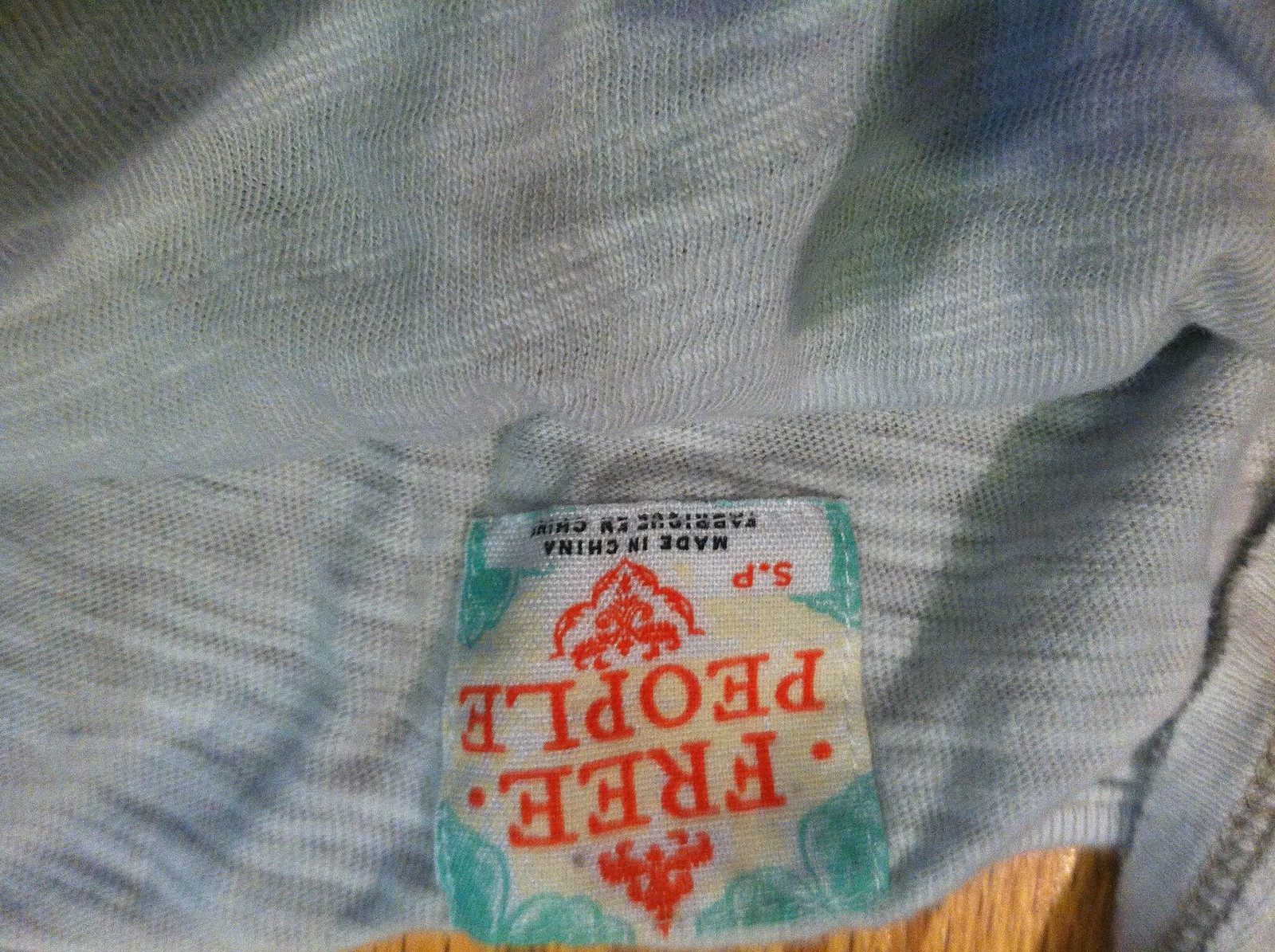The image displays a close-up of a gray, cotton-type shirt from the brand Free People, casually laid out on a wooden tabletop. The shirt features a sewn-in, off-white label with a green cast, bordered with a design resembling treetops. The label prominently displays the brand name "Free People" in orange lettering, flanked by pointy decorations above and below. Additionally, the space around the orange text includes aqua details. Below the brand name, the label reads "Made in China," with further details in another language mostly obscured by a line of thread sewn through them. The hem stitching on the shirt's sleeve is visible, and the item is casually gathered in a pile.